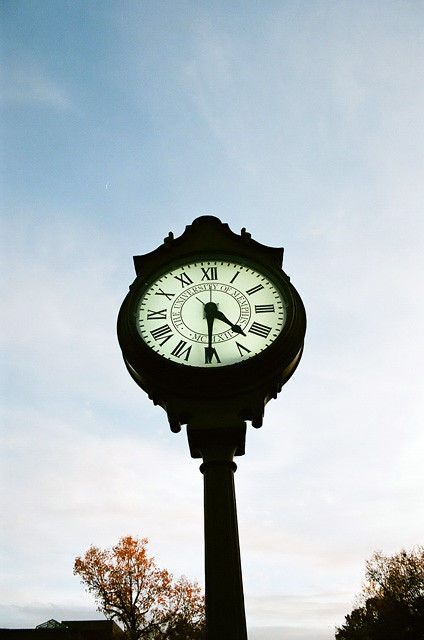A striking outdoor clock stands proudly against a backdrop of a vibrant blue sky adorned with wisps of white clouds. The sky gently fades to near-white as it approaches the horizon, where delicate streaks of pink add a soft touch. To the left of the clock's robust metal pole, a tree with golden and orange leaves adds a splash of autumnal color, while another tree stands gracefully to the right.

The clock itself is the undeniable focal point of the scene. Mounted on a wide metal pole, it features an ornate design with intricate metalwork at its top and bottom, adding a touch of elegance and character. The circular clock face is white and prominently displays Roman numerals from I to XII. The clock hands, including the hour, minute, and possibly a second hand, are black, standing out sharply against the white background. The time reads 4:30.

Adding to its uniqueness, the clock bears the inscription "University of Memphis," indicating its notable location. Below this inscription lies another small Roman numeral, contributing further to the clock's detailed craftsmanship. The entire composition exudes a timeless charm, blending natural beauty with human artistry.